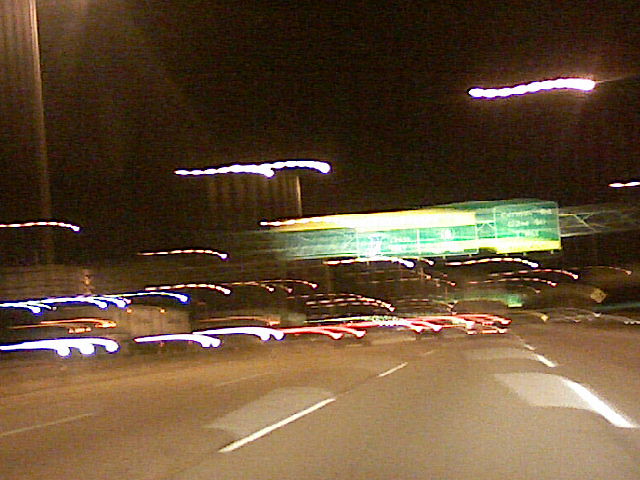The image captures a nighttime, long-exposure photograph of a freeway in the U.S., displaying multiple lanes of traffic headed in both directions. The camera appears to be positioned inside a vehicle traveling in one of the middle lanes. Red taillights from the vehicles ahead stretch into luminous lines due to the motion blur, indicating the direction of travel. On the left side, white headlights from oncoming traffic create similar streaks, suggesting vehicles are moving toward the camera. Over the road, overhead green signs with indistinguishable text and yellow trim mark the lanes and destinations. Blurred yellow streetlights add to the ambient urban lighting, with a hint of tall buildings barely visible behind an overpass or steel structure supporting the signs. The overall effect is a vivid, albeit blurry, representation of a bustling freeway at night.